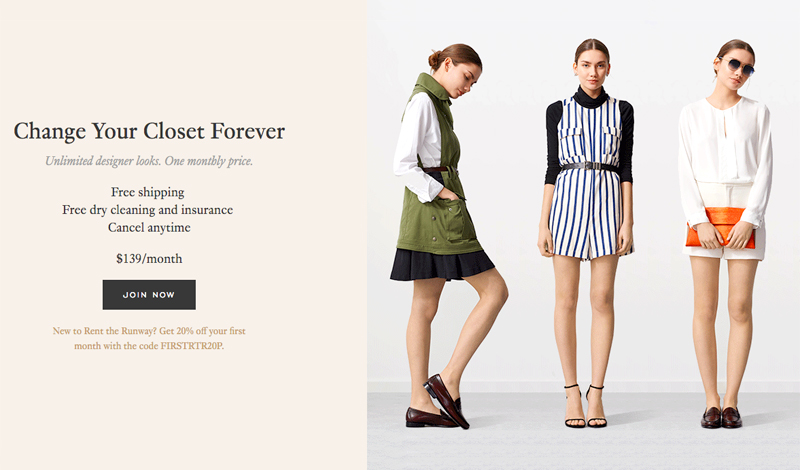On the left side of the image, there is a rectangular section with a very light pale pink background, almost with a beige tint to it. At the top center, in black Times New Roman font, it reads: "Change Your Closet Forever." Below this, in smaller italicized gray text, it states: "Unlimited designer looks. One monthly price." Continuing underneath in the same font as the main header but smaller, it says: "Free shipping," followed by "Free dry cleaning and insurance," and on the next line, "Cancel any time."

Further down, in the same font, it indicates: "$139/month." Beneath this, there is a black rectangle with the capitalized text "JOIN NOW" in the middle, written in a rounded sans-serif white font. Below this button, in a very small light brown font, it reads: "New to Rent the Runway? Get 20% off your first month with the code FIRSTRTR20."

To the right side of the image, there are three women each showcasing different outfits. The first woman is facing slightly to the right with her right arm in her pocket. She is wearing a green dress styled like a vest with black trim, paired with brown loafers. Her hair is tied in a bun.

The second woman, in the middle, is wearing a striped dress cinched at the waist with a black belt, complemented by strappy black shoes. She has dark brown hair pulled back and is wearing earrings. Her hands hang down by her sides.

The third woman on the right is dressed in a white flowy garment that could either be a dress or shorts, holding an orange handbag. She is wearing tortoise-shell sunglasses with shades of brown and beige. Her light brown hair is parted in the middle.